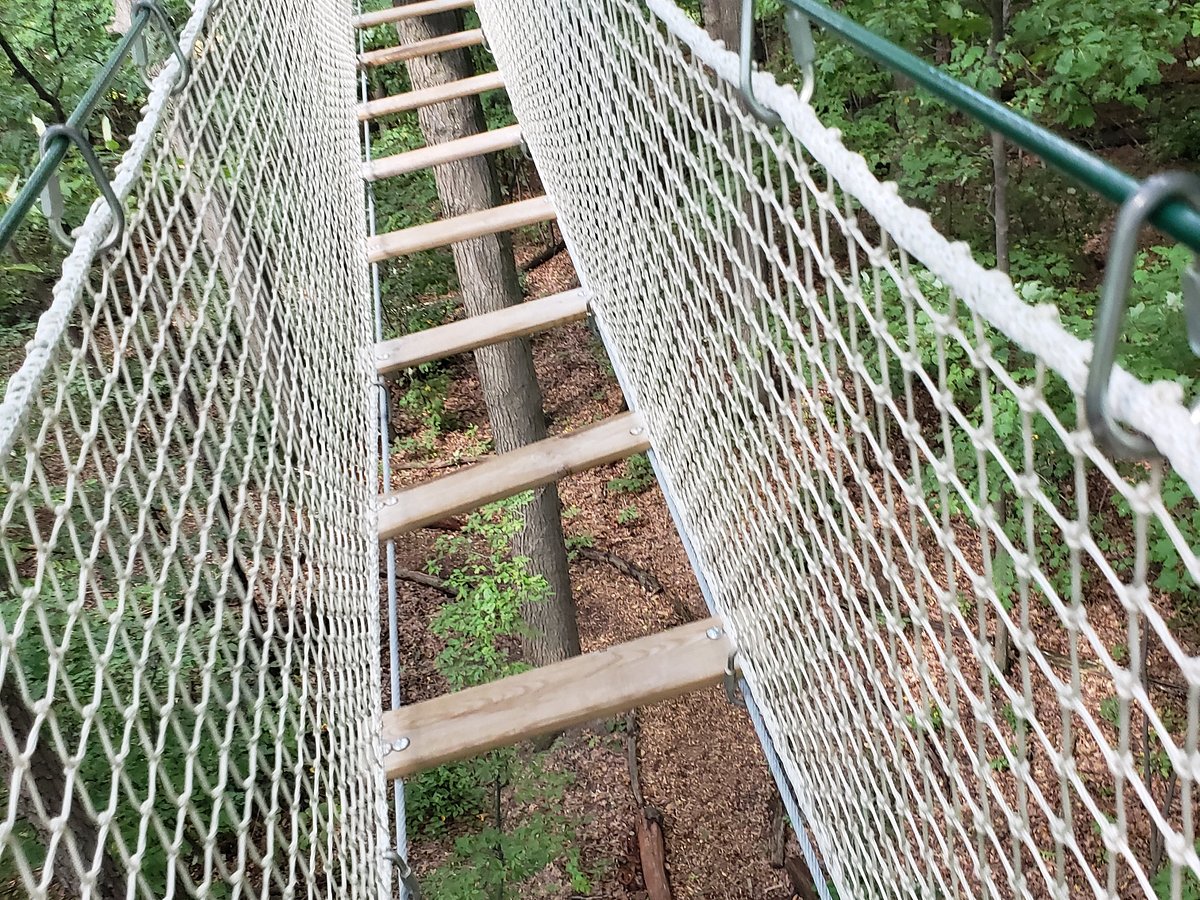The image depicts a suspended rope bridge from a first-person perspective, looking down through the widely spaced wooden planks to the forest floor below. The wooden planks, each placed about a foot apart, create an airy and challenging path. The bridge is suspended high above the ground, about 15 feet, giving it the appearance of a sky bridge amidst a lush forest filled with green leaves and a forest floor carpeted with dead leaves. The railings consist of sturdy metal cables, to which a safety net made of white mesh, resembling a soccer net, is clipped using carabiners. These metal cables run along both sides of the bridge, providing stability and safety. The overall setup resembles a horizontal rope ladder, creating an adventurous ropes course-like obstacle suspended between the trees.